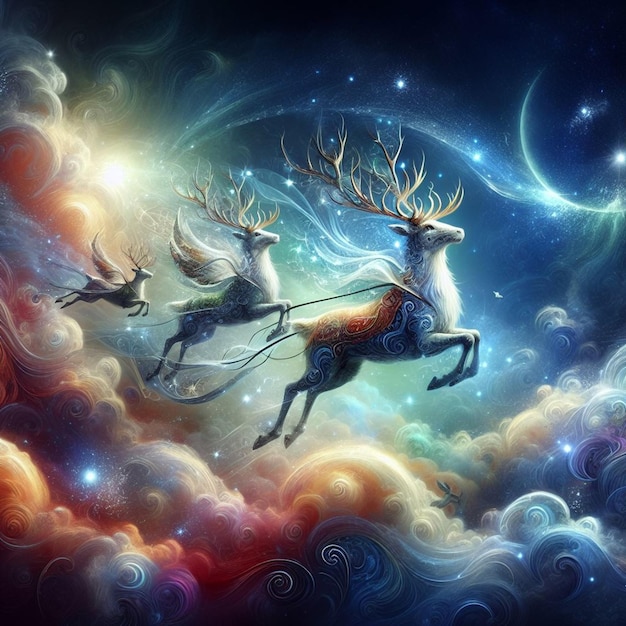The image resembles a fantastical scene from a novel, featuring three cosmic reindeer-like creatures flying through a vibrant, swirling sky. The creatures, amalgamations of deer, pegasus, and unicorn, have massive, bright yellow antlers with 30-40 points and exhibit a gradient of rainbow hues. The largest is in the front, with the second and third progressively smaller, connected as if pulling an unseen sleigh. Their hides glimmer with blue and mechanical-like swirls, and the back two have wings.

The sky is a mesmerizing array of pastel colors and swirling clouds, ranging from dark blue waves at the bottom to orange and red swirls on the left. The right upper corner showcases a navy blue moon or planet surrounded by bright star-like dots. Additionally, there’s a glowing sun in the top left corner. The entire scene is computer-generated, giving it a cosmic, surreal, and dream-like quality, with no text to distract from the spectacle. The image is clear and highly detailed, capturing a mystical moment in a vividly lit sky.